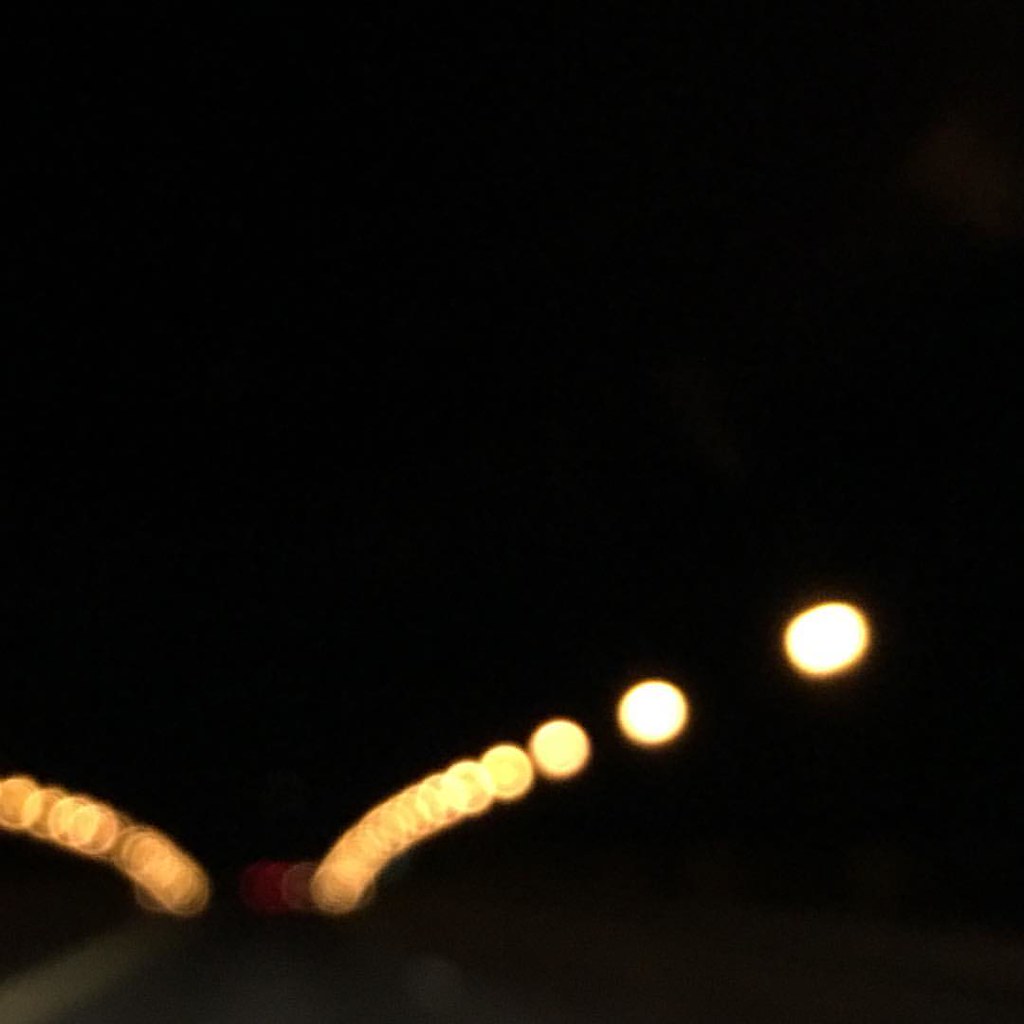This photograph, captured outdoors at nighttime, portrays a scene dominated by a series of blurry, orange-hued lights extending along what appears to be a road. The image is indistinct, with the lights blending together into a continuous, hazy streak that suggests movement or a long exposure shot. In the bottom left corner, faint road lines can be discerned, offering the only concrete clue to the setting. The overall impression is one of obscured details and ambient nighttime ambiance, with the focus on the luminous trail of lights marking the path of the road.